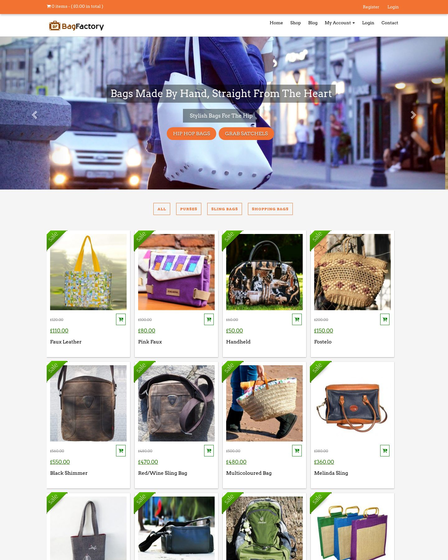This image showcases the landing page of the Bagfactory website in rich detail. At the top, an orange stripe runs across the screen, featuring "Register" and "Login" options on the right side. Directly below, a sleek white menu bar is displayed. On the left of this menu bar is the Bagfactory logo and name; "Bag" is styled in brown, while "factory" is in black. The menu options are aligned to the right and include: Home, Shop, Blog, My Account (with a downward arrow), Login, and Contact.

Dominating the page is a slider photograph capturing a scene of a chic woman crossing a busy street. She carries a white leather tote bag over her shoulder, with background elements including pedestrians standing against buildings and a white van to her left. A bold black box overlays the image with the text: “Bags made by hand straight from the heart.” Below this, two prominent orange buttons read "Shop Bags" and "Grab Satchels."

Further down the page, four tags are displayed: All, Price, Fling Bags, and SA Shopping Bags. Beneath these tags are 16 individual images of various bags. Each bag is housed within its own box, accompanied by a green slanted banner at the top left corner, indicating key information such as the price and the name of the bag. The bags are diverse, featuring mostly tote bags and satchels. Noteworthy mentions are the top right image, showcasing a weaved tote bag, and the bottom right image presenting a set of three wicker bags with gold handles. The background of this section is clean and white, providing a crisp contrast to the vibrant product displays.